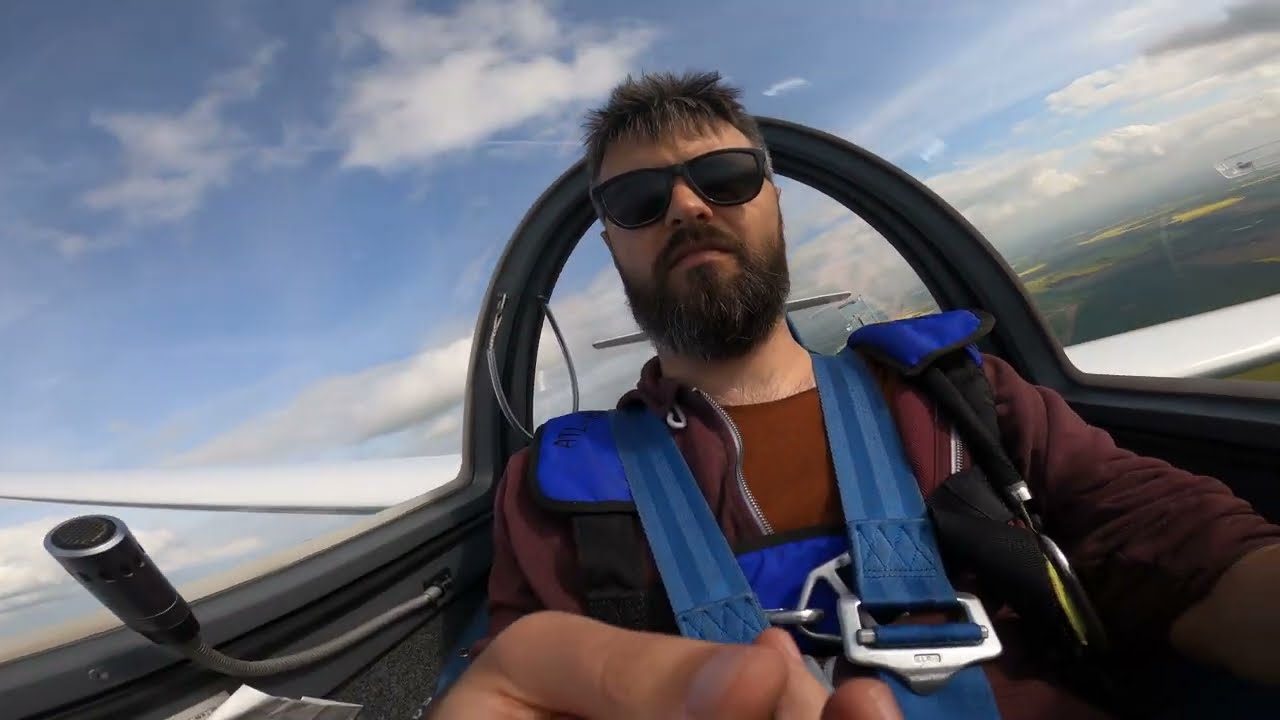In this striking aerial selfie, a man, comfortably secured with blue shoulder straps in what appears to be a high-speed aircraft, captures the moment. He sports a red shirt beneath a maroon zip-up hooded sweatshirt, complemented by sunglasses and a dark, full beard that connects seamlessly with his short, spiky hair. With a confident outstretched hand, likely holding a phone to snap the photo, he appears engrossed in his surroundings. Behind him, through the aircraft's window, a beautiful expanse of a vibrant blue sky dotted with fluffy white and gray clouds unfolds. Below, a patchwork of green fields and grasslands stretches out, providing a stunning contrast to the clear skies. The aircraft wings are faintly visible on either side, suggesting a slight tilt of the plane and adding a dynamic sense of motion to this high-quality image.